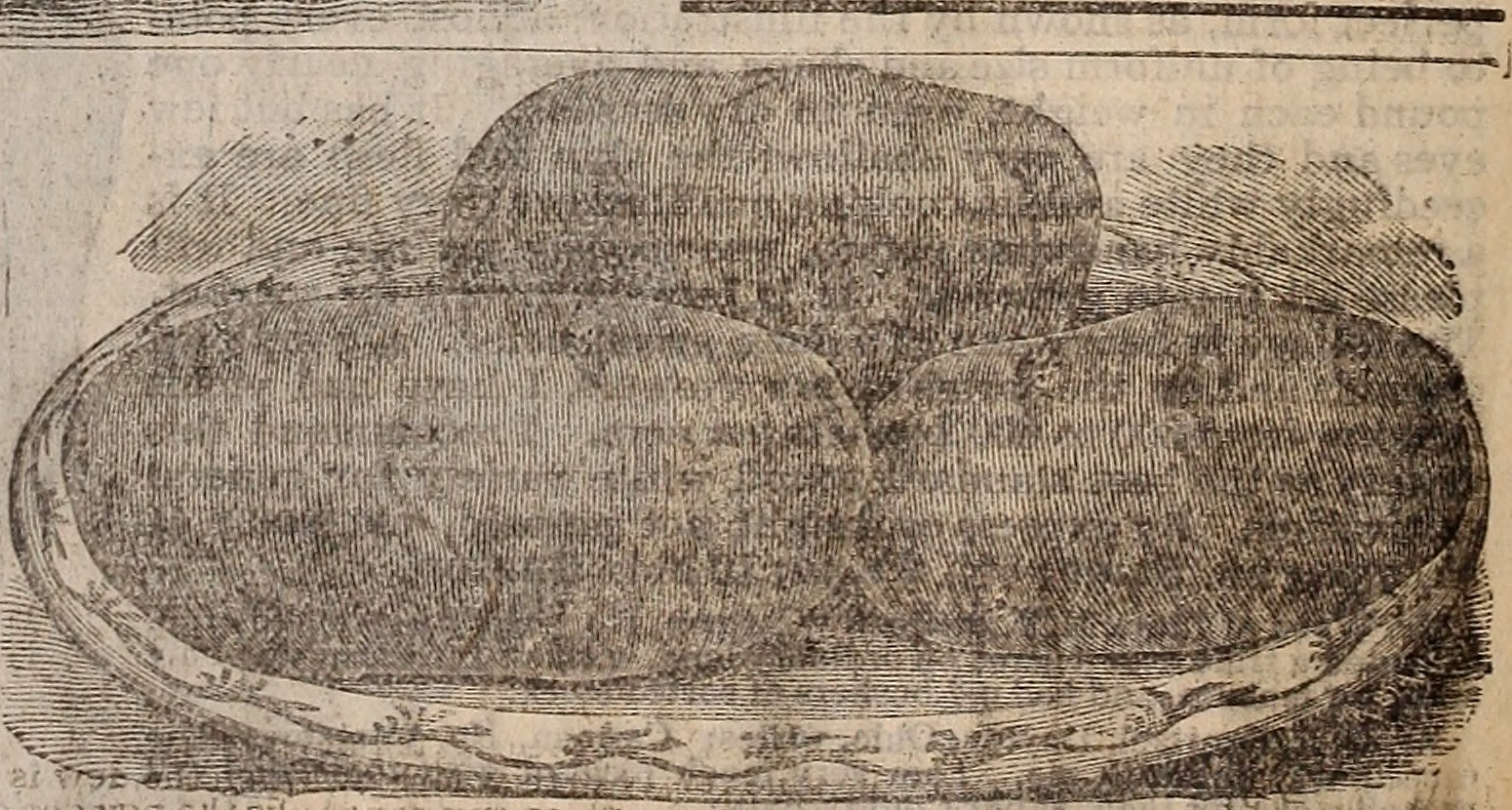This horizontal, rectangular image depicts a cream-colored piece of paper featuring a detailed drawing in black lines. The primary focus is a tray or plate occupying the entire bottom portion of the picture, adorned with intricate black lines along its border, resembling a thumbprint or fingerprint pattern. Inside the tray sit three russet baked potatoes, each uniquely shaped. The left potato is oval and long, the right one is slightly shorter with visible eyes, and a third potato rests in the background. The design extends to include elements that appear like branches or trees on either side of the tray, contributing to the overall ancient, almost Egyptian or pyramidal aesthetic of the drawing.